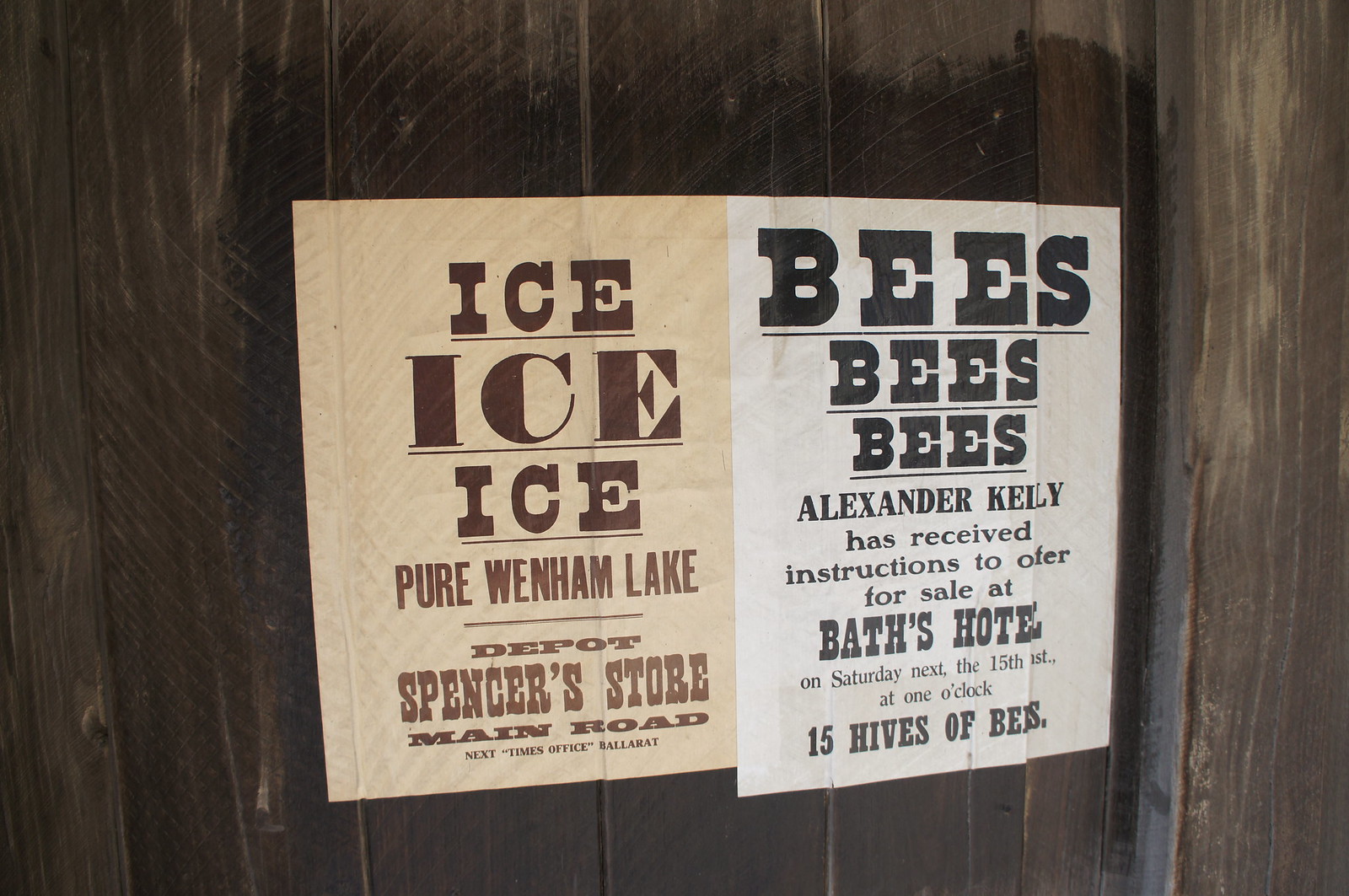The image showcases two paper signs affixed to a dark brown wooden plank fence. The sign on the left features an off-white background with bold brown text at the top reading "ICE, ICE, ICE," repeated three times. Beneath this, in smaller brown text, it states "Pure Wenham Lake," followed by "Depot, Spencer's Store, Main Road." At the bottom, the text reads "Next, Times Office, Ballarat." The sign on the right is on white paper with large, bold black text at the top that says "BEES, BEES, BEES," repeated three times. Below that, in standard black text, it details, "Alexander Kelly has received instructions to offer for sale at Baths Hotel on Saturday next, the 15th at 1 o'clock, 15 hives of bees."